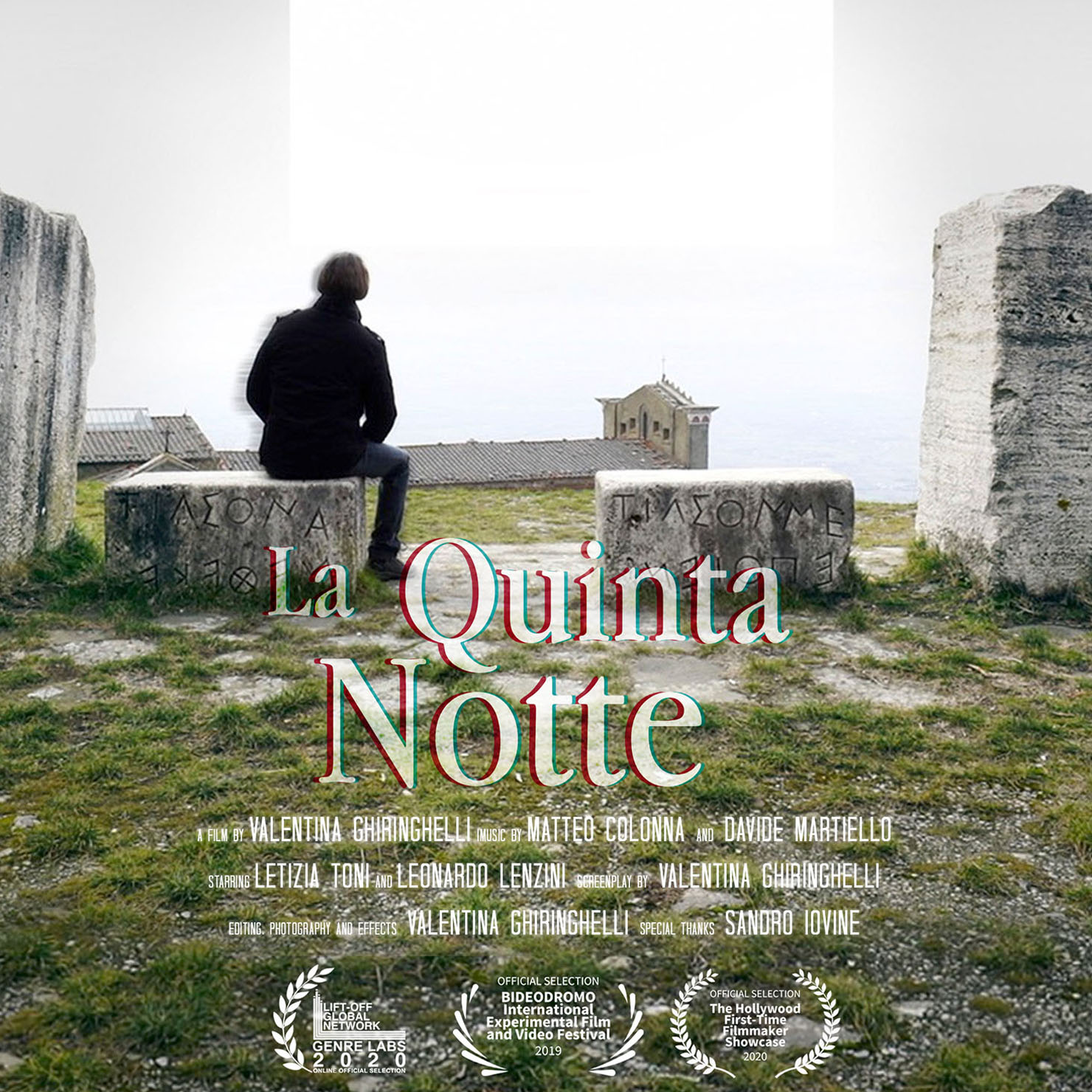The image is a detailed movie cover for the film "La Quinta Notte." The background is filled with a gray sky above a faint, almost ghostly body of water. At the focal point is a man with short brown hair, dressed in a black jacket and blue jeans, sitting with his back to the viewer on one of two grayish-brown stones, both carved with different symbols. Next to him lies another stone with more engravings, looking like old, irregularly shaped tombstones. On either side of these stones stand two larger stones of a similar hue, giving the scene an ancient, somber feel. The man's gaze is focused on the water before him, adding a contemplative atmosphere to the image. The title "La Quinta Notte" is prominently displayed across the center in large white letters outlined in red. Credits below indicate the film is by Valentina Ghirangeli, with music by Matteo Colonna and David Martiello, listing the starring actors' names. At the bottom, accolades are mentioned, including the Liftoff Global Network Genre Labs 2020, the Bernanetto International Experimental Film and Video Festival 2019, and the official selection of the Hollywood First Time Filmmaker Showcase 2020.